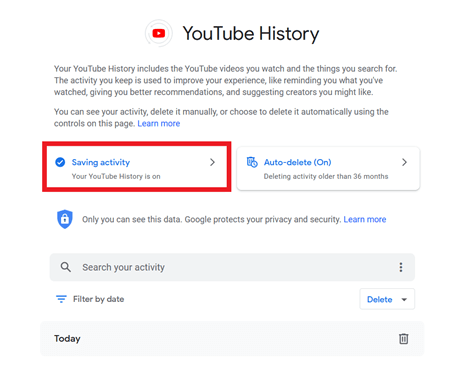The image features the YouTube logo prominently at the top. Below the logo, in bold black letters, the text "YouTube History" is displayed. Underneath this header, in smaller black font, a detailed paragraph outlines the function and benefits of YouTube history. The paragraph explains that your YouTube history includes both the videos you watch and the searches you perform. It highlights that this activity data is utilized to enhance your experience by reminding you of what you've viewed, offering improved recommendations, and suggesting new creators you might enjoy.

The paragraph continues after a line break, informing you that you have the ability to view, manually delete, or set up automatic deletion of your activity through the controls provided on this page. A blue hyperlink labeled "Learn more" is included for additional information.

Below the explanatory text, there is a white box labeled "Save an activity," which includes a check mark within a blue-bordered box. Directly beneath this, in black text, it states: "Your YouTube history is on." To the right of this section, another box features blue text indicating "Auto-delete on." Beneath this, the text specifies that any activity older than 36 months will be automatically deleted.

Finally, a privacy note at the bottom assures users that only they can see their data, and that Google takes measures to protect their privacy and security.